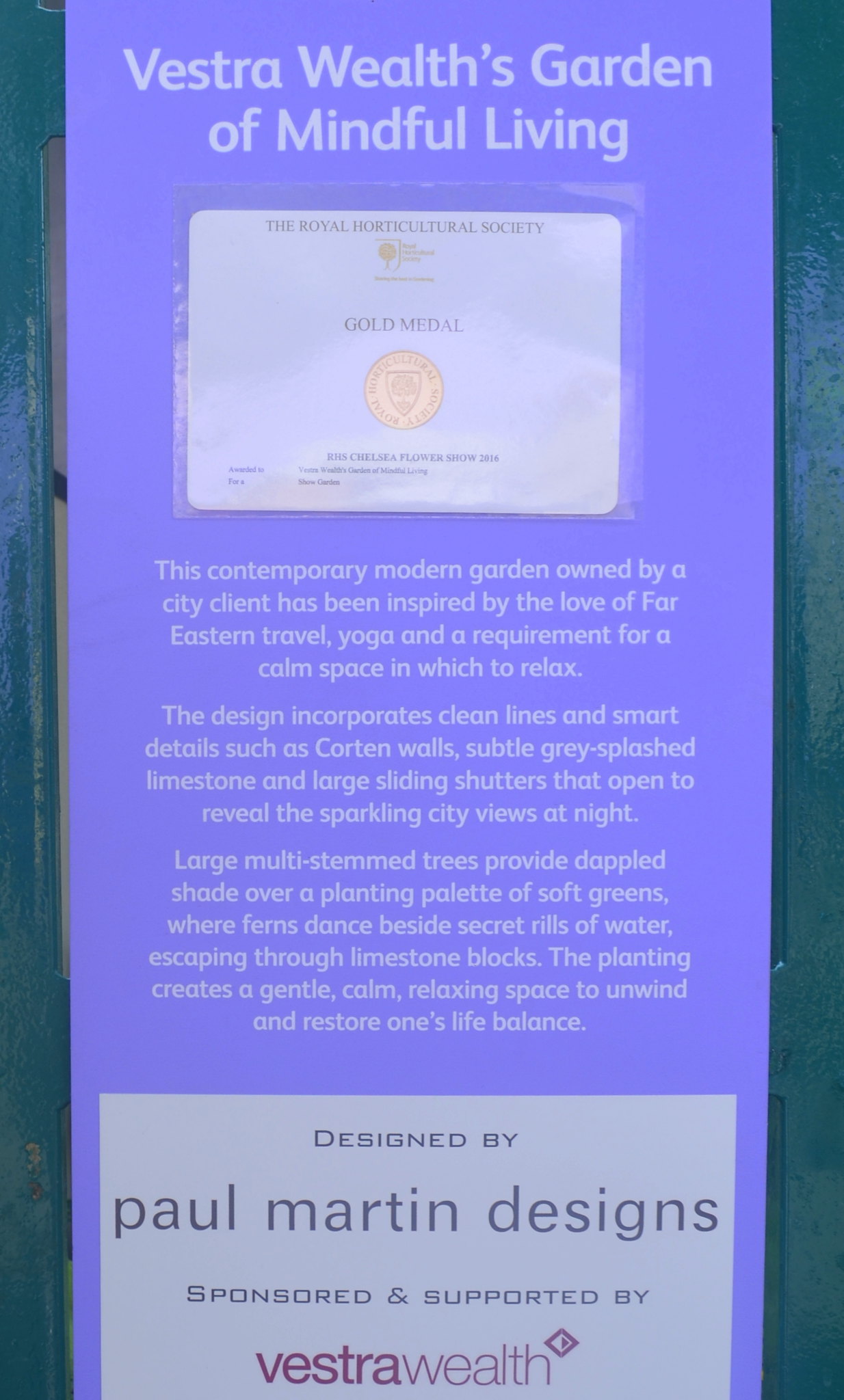The image is an advertisement for the Vastra Women's Garden of Mindful Living program, set against a purple background with white text. At the top, it reads "Vastra Women's Garden of Mindful Living." Below this is a white rectangle featuring the Royal Horticultural Society's Gold Medal emblem, with a gold-colored coin and some small, unreadable text beneath it. The main body of the poster details the serene and thoughtfully designed garden: "This contemporary modern garden, owned by a city client, has been inspired by the love of Far Eastern travel, yoga, and the need for a tranquil space to relax. The design incorporates clean lines and sophisticated details such as corten walls, subtle gray-splashed limestone, and large sliding shutters that open to reveal the sparkling city views at night. Large multi-stemmed trees provide dappled shade over a planting palette of soft greens, where ferns coexist with secret rills of water flowing through limestone blocks. The planting fosters a gentle, calm, and restorative space to unwind and restore one's life balance." At the bottom, the poster credits the design to Paul Martin Design and notes that it is sponsored and supported by Vestra Wealth.